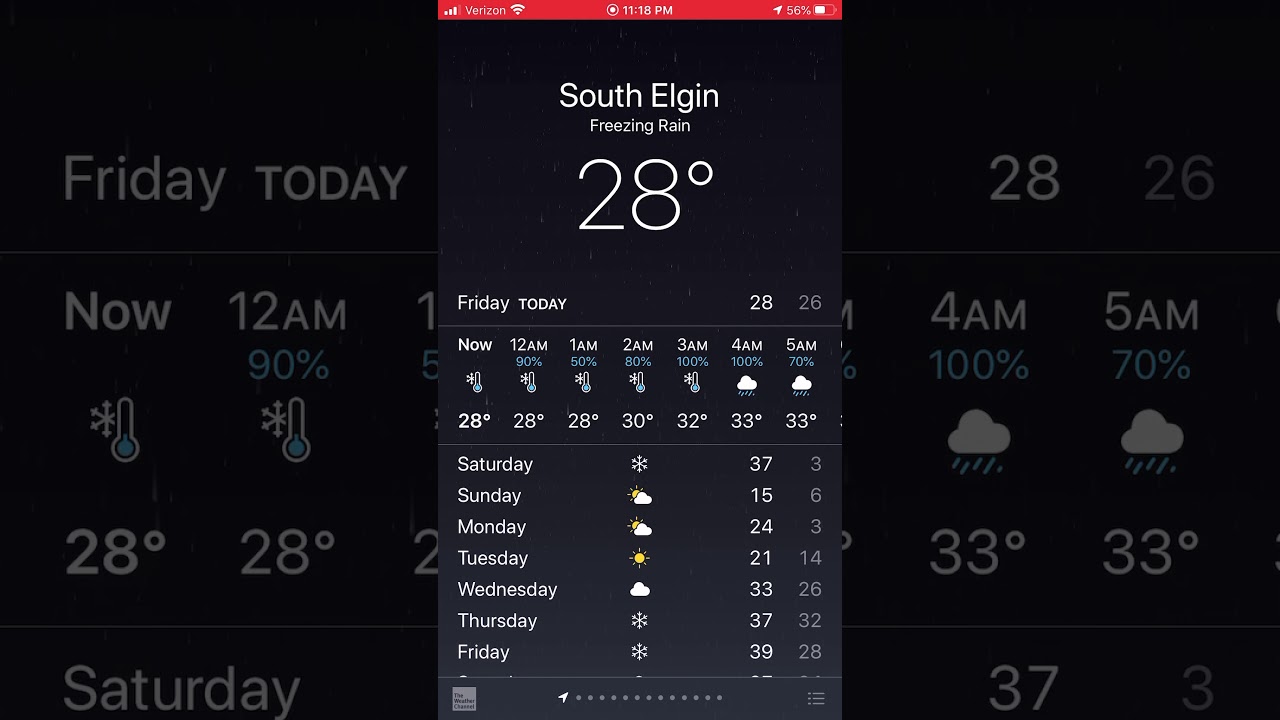The image is a screenshot featuring a vertically oriented rectangular central box set against a horizontally extended black background. The main display shows various status icons at the top: "Verizon" carrier signal, Wi-Fi connection, the time "11:18 p.m.," and a battery status at "56% charged." Below these indicators, the screen presents a weather update for "South Elgin," indicating "freezing rain" and a current temperature of "28 degrees." The date and day are listed as "Friday, 28th."

The detailed weather forecast includes temperature readings by the hour: showing 28 degrees at 12 a.m. and 1 a.m., 30 degrees at 2 a.m., 32 degrees at 3 a.m., 33 degrees at 4 a.m. and 5 a.m. Further down, a weekly overview provides daily forecasts for Saturday through Friday, displaying weather icons and anticipated high and low temperatures. The icons indicate conditions like snow or rain, with a temperature gauge and relevant symbols (such as a cloud with showers) showing for specific times like 4 a.m. and 5 a.m. The background screen is a zoomed-in view of the hourly temperature forecast, mirroring the detailed temperature and weather information presented in both displays.